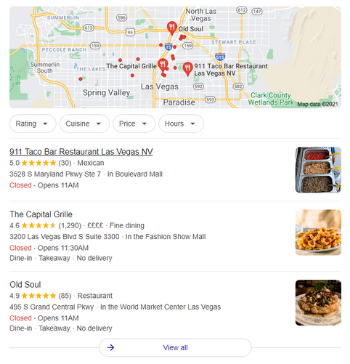This screenshot depicts a user interface displaying a search for restaurants near Las Vegas. At the top of the image is a map pinpointing locations of various eateries. The map highlights North Las Vegas and features three red icons, each marked with a knife and fork, indicating restaurant locations. 

The icons correspond to three specific restaurants: "Old Soul" at the top, "Capital Grill" in the middle, and "9-1-1 Taco Bar Restaurant Las Vegas" at the bottom.

Below the map, the screen displays four navigational tabs labeled "Rating," "Cuisine," "Price," and "Hours." These tabs likely allow the user to filter restaurant search results based on these criteria.

Further down, the detailed information of the three highlighted restaurants is provided:

1. **9-1-1 Taco Bar Restaurant Las Vegas**:
   - Rating: 5 stars
   - 30 reviews
   - Cuisine: Mexican

2. **Capital Grill**:
   - Rating: 4.6 stars
   - 1,290 reviews
   - Cuisine: Fine Dining

3. **Old Soul**:
   - Rating: 4.9 stars
   - 85 reviews
   - General Category: Restaurant

All these restaurants are located in the Las Vegas area, providing potential dining options for the user.